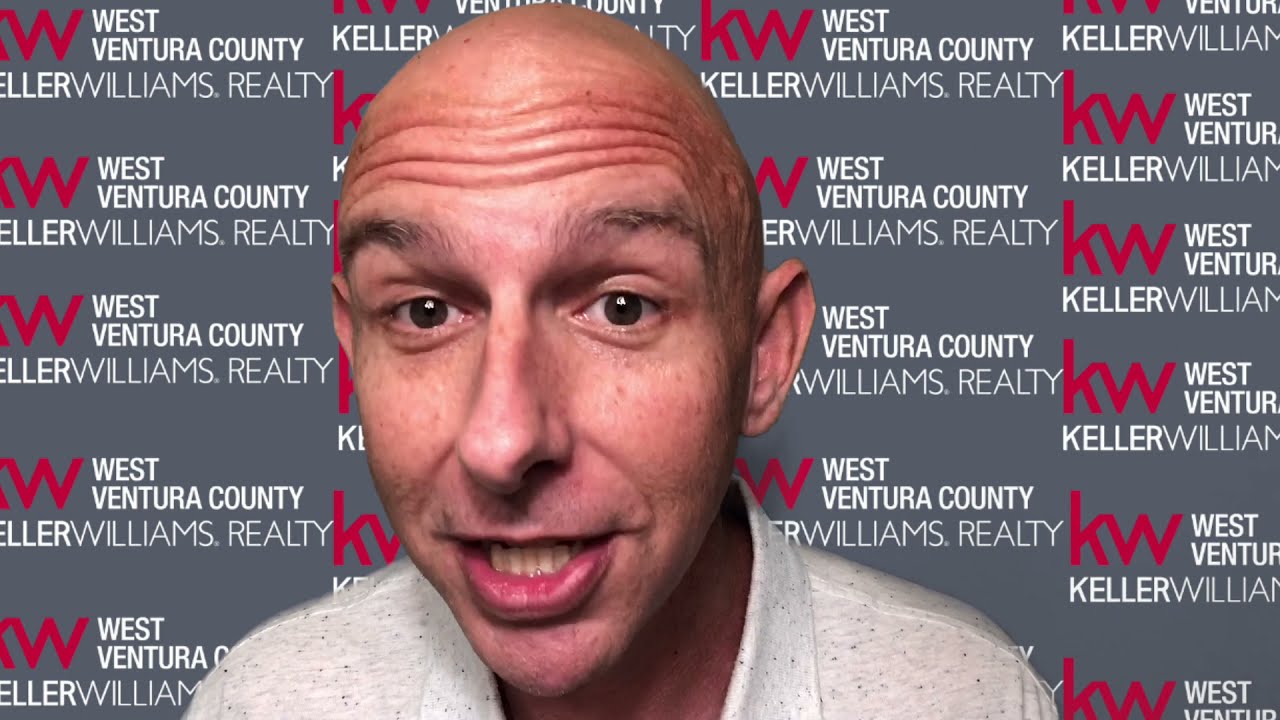In this zoomed-in image, a bald, Caucasian man with pronounced forehead wrinkles and black, curvy eyebrows is prominently featured. He has freckles and is wearing a light heather gray collared shirt with small black dots. His mouth is open, revealing his lower teeth, and he appears to be speaking. The man is centered against a grey backdrop featuring a repeating company logo. This logo consists of a large red "KW" with "West Ventura County" in smaller white text to the right, and "Keller Williams Realty" below in white capital letters. The logo pattern spans the background in four columns and five rows, giving the impression of a branded setting, possibly for a video or presentation.